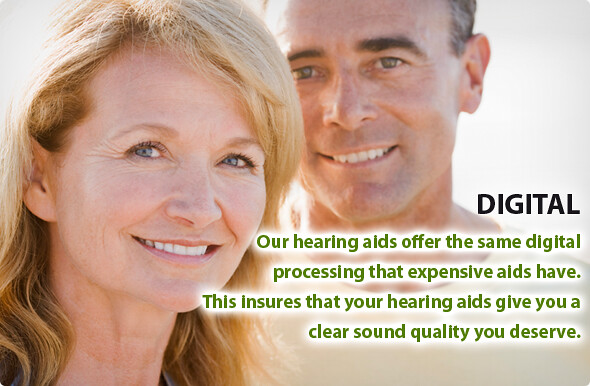The advertisement features a vibrantly smiling woman with long blonde hair and blue eyes, displaying subtle smile lines near her eyes. She is positioned on the left side of the image, slightly in front of a man who stands to her right. The man has darker gray hair, bluish eyes, and a similarly warm smile. They both appear to be in their 40s or 50s, exuding an inviting and relatable aura. The background is white with a hint of tan, illuminated as if the sunlight is shining from behind them. The ad text is strategically placed below the man's chin, with the word "Digital" emphasized in bold black letters. Beneath it, in green text with a white glow, it reads: "Our hearing aids offer the same digital processing that expensive aids have. This ensures that your hearing aids give you the clear sound quality you deserve." This clean, bright setting effectively underscores the advanced digital quality of the hearing aids being advertised.